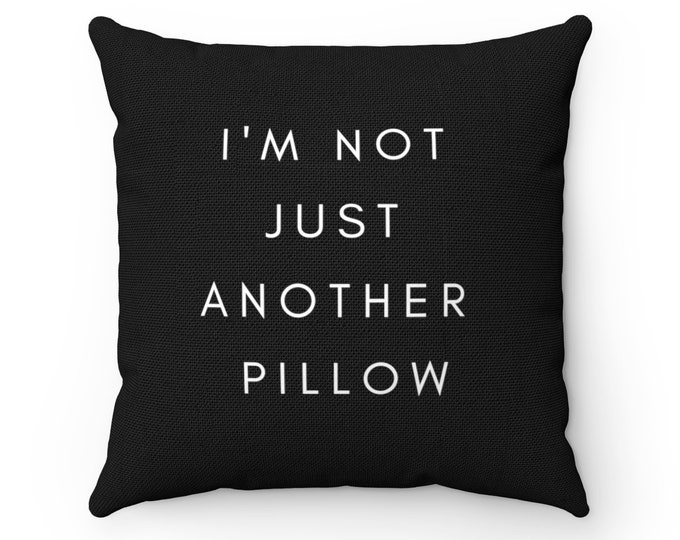The image features a large, square-shaped black pillow at the center against a plain white background. The pillow, which appears finely textured and possibly knitted, has pointed and pronounced corners. In the center of the pillow, there are four lines of text in bold, white capital letters with generous spacing between each letter. The text reads, "I'M NOT JUST ANOTHER PILLOW," and is perfectly centered both horizontally and vertically. The overall design is professional, with a subtle shadow detectable along the bottom and right sides of the pillow, giving it a clean and advertised look.